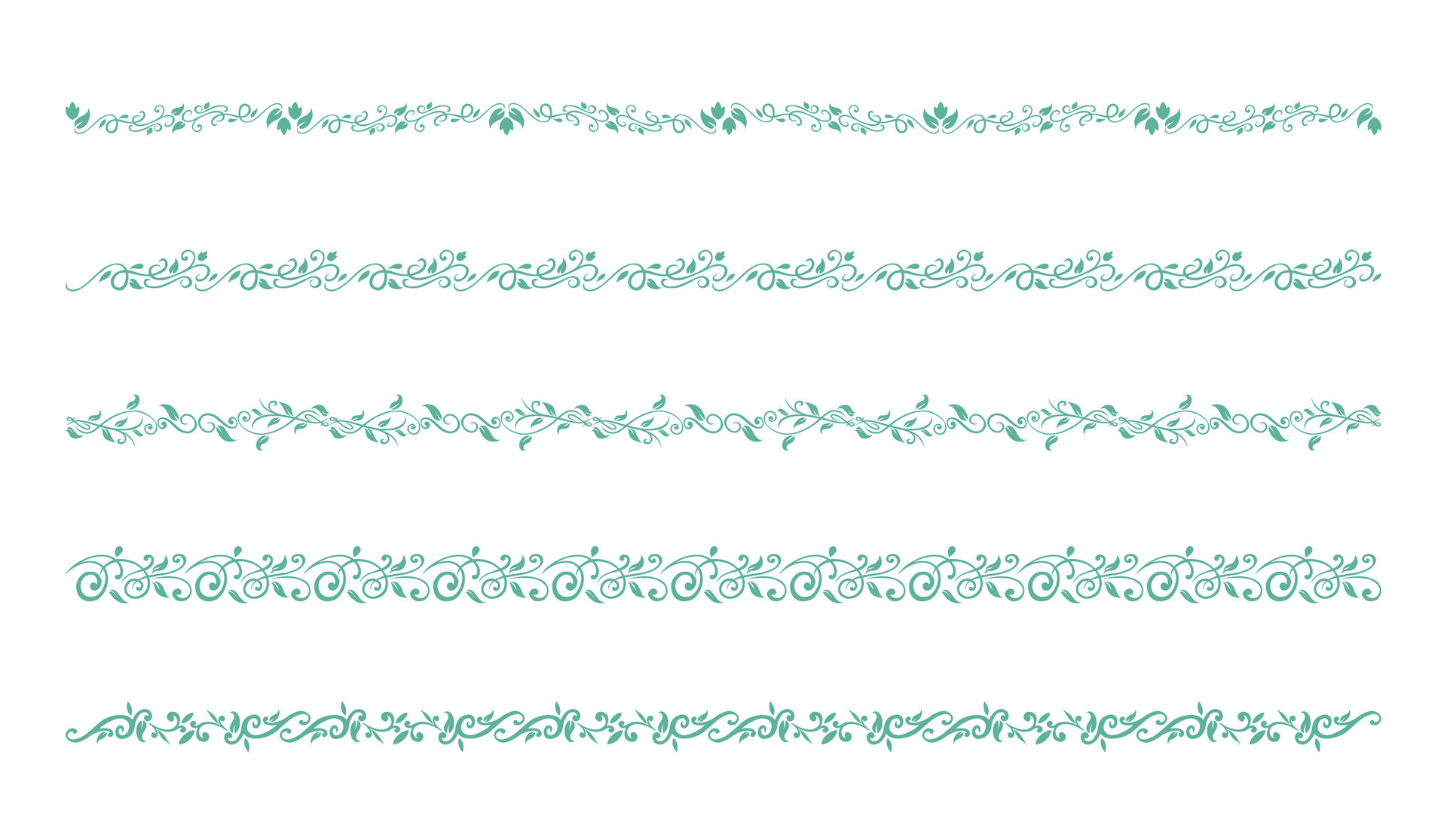The image features five delicate borders arranged horizontally, each crafted with fine bluish-green ink. The ornate, intricate designs are reminiscent of leaves and vines, flowing elegantly in a pattern that almost suggests cursive handwriting. Every line is unique, with no two designs exactly alike, enhancing the natural, organic feel of the artwork. The plant-like motifs give the impression of something that could adorn the edges of an embroidery or frame a picture, adding a touch of nature-inspired beauty to any bordered space. The detailed, swirling fashion of the lines creates a visually captivating effect that is both charming and sophisticated.